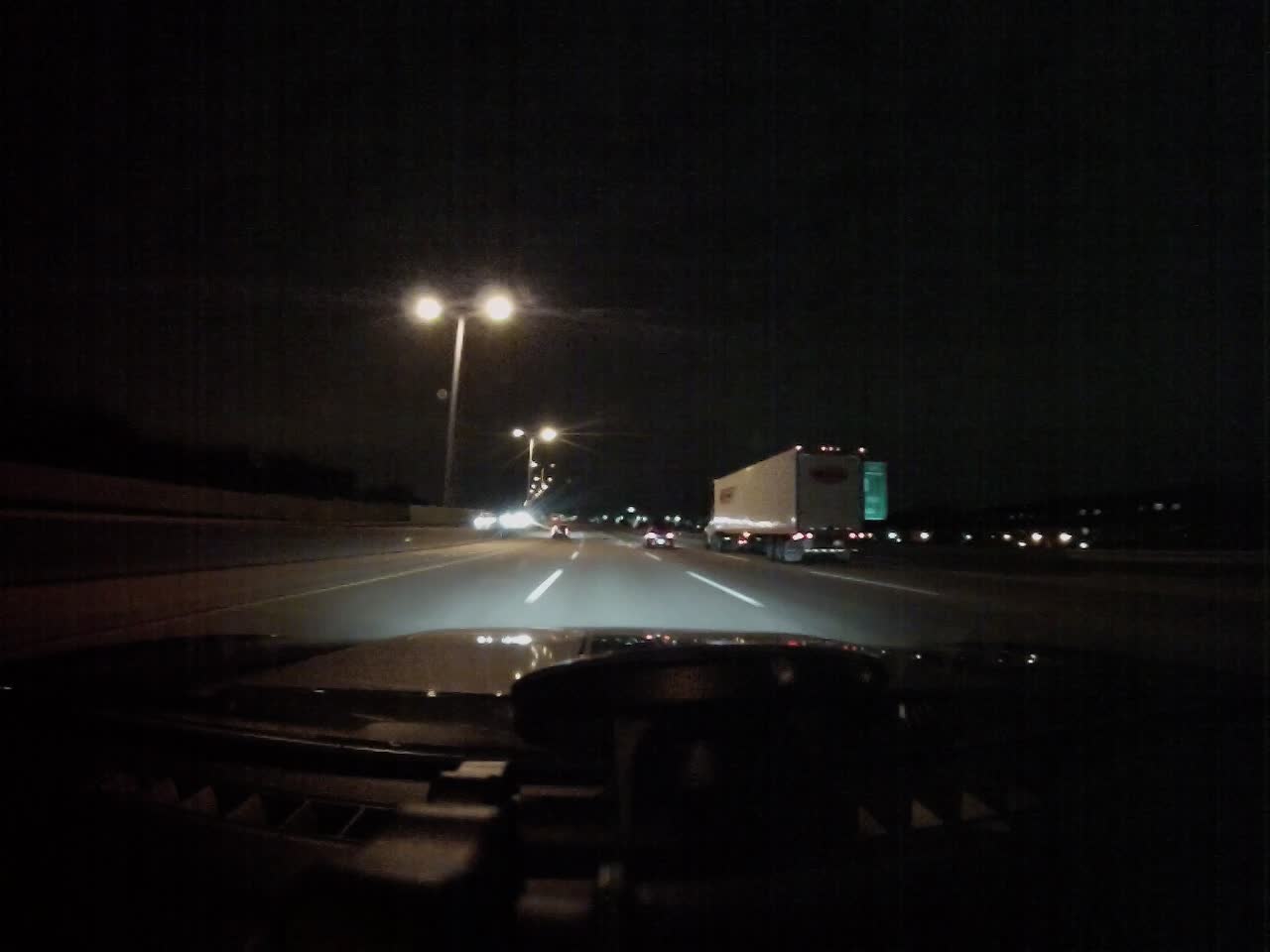This image captures a serene evening drive along a four-lane interstate highway, likely filmed from a dashboard camera. The highway is illuminated by streetlights, casting a gentle glow on the scene. A large tractor-trailer dominates the foreground, partially obscuring a road sign, which adds an element of mystery about the location. To the right, the silhouette of another vehicle is visible, while cars approach from the left-hand lanes, suggesting a steady but not overwhelming flow of traffic. The sky above is darkening, hinting at the transition from twilight to night. The surroundings lack significant urban structures, indicating a rural area or a stretch of the interstate bordered by open fields, rather than a bustling cityscape.